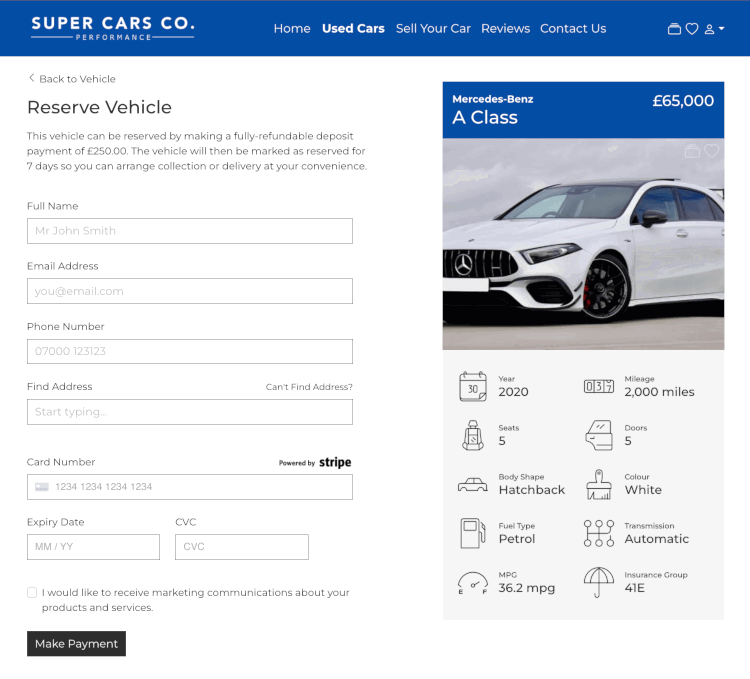Screenshot Description: Supercars Website - Reserving a Mercedes-Benz A-Class

The screenshot captures a webpage from the Supercars Company website, specifically focusing on the "Used Cars" section. The website is well-organized with navigation options such as Home, Used Cars, Sell Your Car, Reviews, and Contact Us. The user is currently on the "Used Cars" page, attempting to reserve a vehicle.

Highlighted is a 2020 Mercedes-Benz A-Class, priced at £65,000, with a mileage of just 2,000 miles. The car is a white hatchback with 5 doors and seating for 5. It boasts an automatic transmission, a petrol engine, and an impressive fuel efficiency of 36.2 miles per gallon. This vehicle falls under insurance group 41E.

To reserve the vehicle, the user is informed that a fully refundable deposit of £250 or €250 can be made. Once the deposit is paid, the car will be marked as reserved for seven days, allowing the user time to arrange for collection or delivery at their convenience.

The reservation process requires the user to fill out a form with fields for their full name, email address, phone number, and address. Payment information, including card number, expiration date, and CVC code, is also needed. The payment system is powered by Stripe, ensuring a secure and convenient transaction.

There is an option to opt-in for marketing communications about the company’s products and services. This can be checked or unchecked based on the user’s preference. Finally, a black button with white lettering labeled "Make a Payment" is present, which the user can click to complete the reservation.